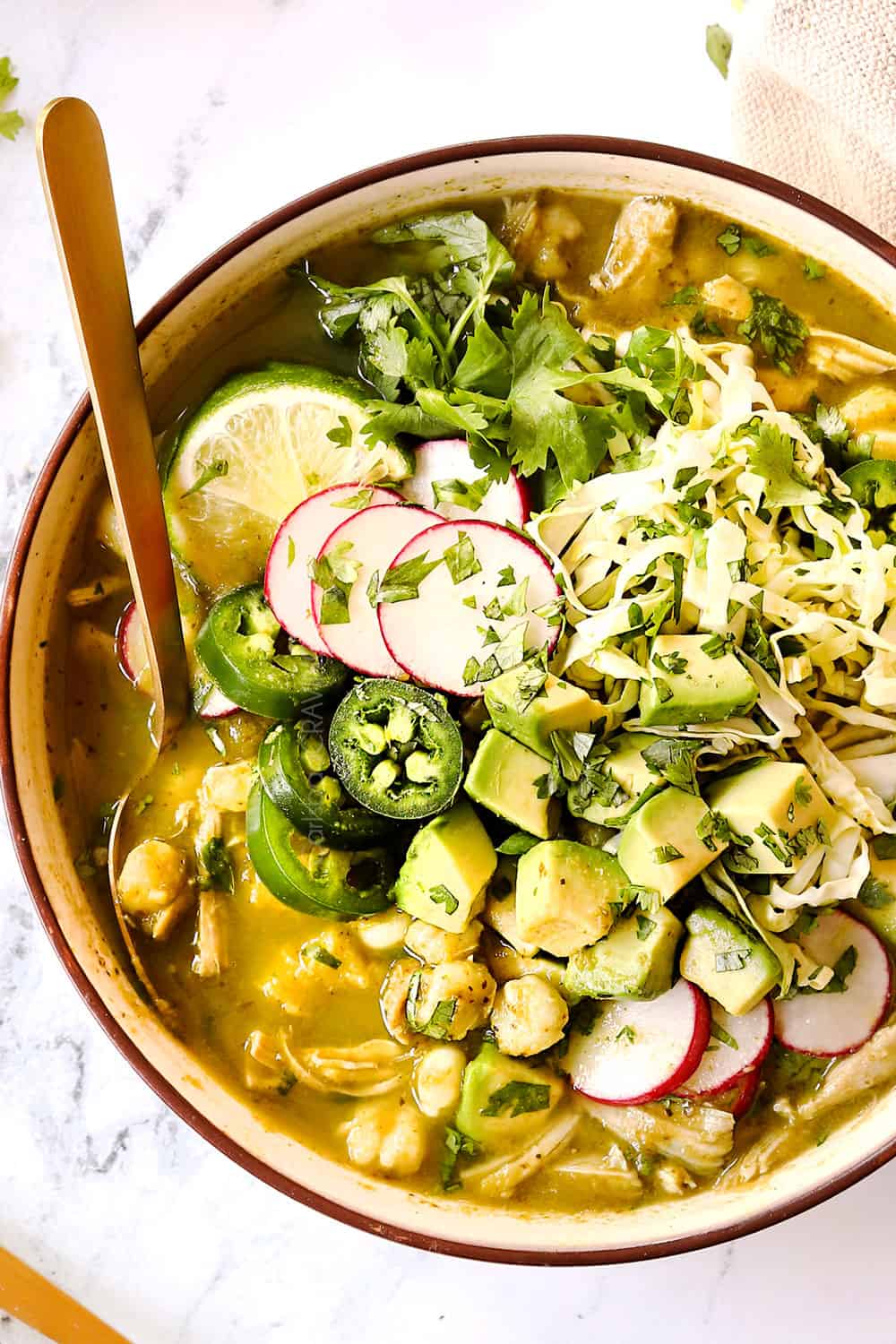This is a detailed photograph of a richly garnished Mexican dish, likely pozole or menudo, served in a white bowl with a deep brown or burgundy rim. The bowl, which is placed on a marble-textured table, contains a hearty stew made with shredded chicken, maize corn, and is topped with an array of colorful and fresh ingredients. Visible toppings include sliced radishes, jalapenos, avocado slices, and a slice of lime. Fresh cilantro and possibly other greens like spring mix or herbs such as parsley or basil are sprinkled across the top, adding vibrant green accents. A prominent gold spoon is placed inside the bowl, slightly protruding to the left. In the top right corner of the image, there's a piece of tan muslin cloth. The stew has a thick consistency with a brownish broth and appears flavorful and inviting.